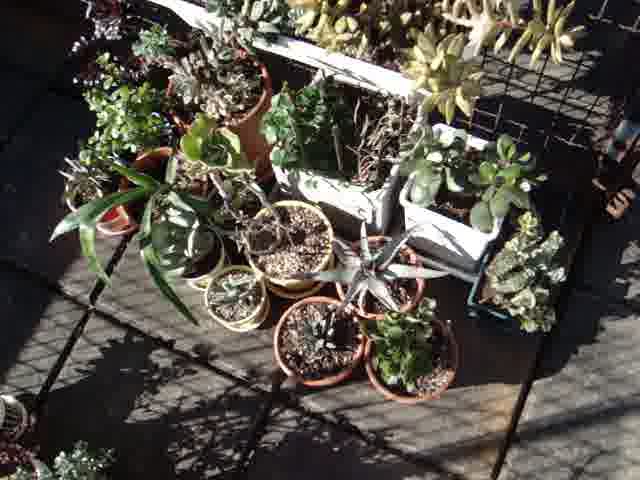The photograph is a top-down view of an outdoor arrangement featuring a diverse collection of potted succulents situated on a deck or paved area with large, square paver stones. The pots, varying in shape and size, include white square pots centrally located, surrounded by more circular pots in shades of orange and yellow. The succulents exhibit a range of forms, from star-shaped and spiky types to those resembling cacti. While the plants near the center have yellow-tinged leaves, those on the left side appear larger, with some having long leaves and others with many short leaves. Shadows cast on the ground suggest that the photo was taken in sunlight, and there is a visible grate in the upper left corner, hinting at additional structural elements. Despite the overall clarity being somewhat compromised, the sunlight highlights the vibrant variety of the succulent collection.